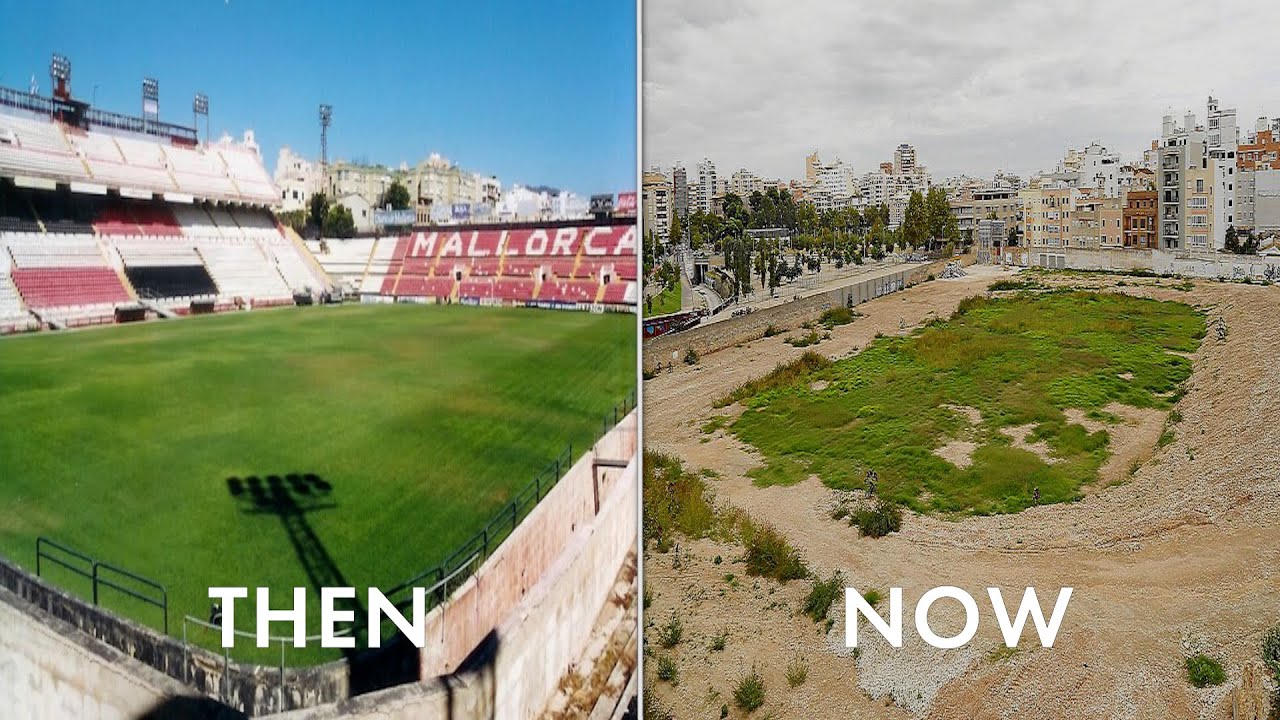In the composite image of a "then and now" scene, the left side depicts a vibrant stadium, likely a soccer or football arena, with two-tiered bleachers in red, white, and black seating. The top of the bleachers spells out "Mallorca" in large red letters. The field is lush green, encircled by concrete, and light towers cast long shadows across the pitch, indicating the sun is setting behind the viewer. The far end of the stadium reveals a cityscape under a clear blue sky, accentuating the overall lively atmosphere.

The right side of the image, labeled "now," starkly contrasts the former view, depicting an empty, desolate lot. The once lively stadium is replaced by a mostly barren landscape with only traces of grass where the field used to be. The ground is smooth gravel, ready for new development. Surrounding skyscrapers and apartment buildings still peek in from the city, but under a cloudy sky, the area's transformation from a bustling stadium to an empty lot is otherworldly.